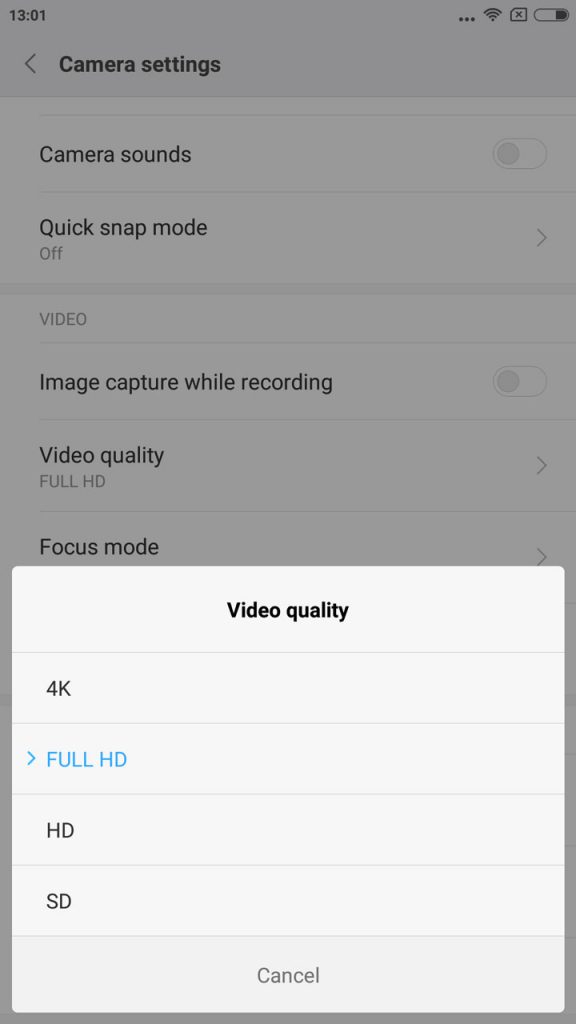The screenshot depicts the camera settings interface of a smartphone, captured at 1:01 p.m., as indicated by the time displayed at the top left corner of the screen ("13:01"). To the right of the time, several icons are visible: the Wi-Fi symbol, a square with an 'X' in it, and the battery icon showing a charge level of just under half.

Below these icons, the main camera settings layout is displayed. The first visible option is "Camera sounds," which is toggled off. Next is "Quick snap mode," also toggled off. The settings continue with a section titled "Video settings." Within this section, "Image capture while recording" is shown to be off, and "Video quality" is set to Full HD.

Partially obscuring the screen, a pop-up window titled "Video quality" presents four selectable options: 4K, Full HD, HD, and SD. The currently selected quality, Full HD, is highlighted in bright blue text, indicating its active status. Due to the pop-up window, the settings for focus mode and any subsequent options are not visible in the screenshot.